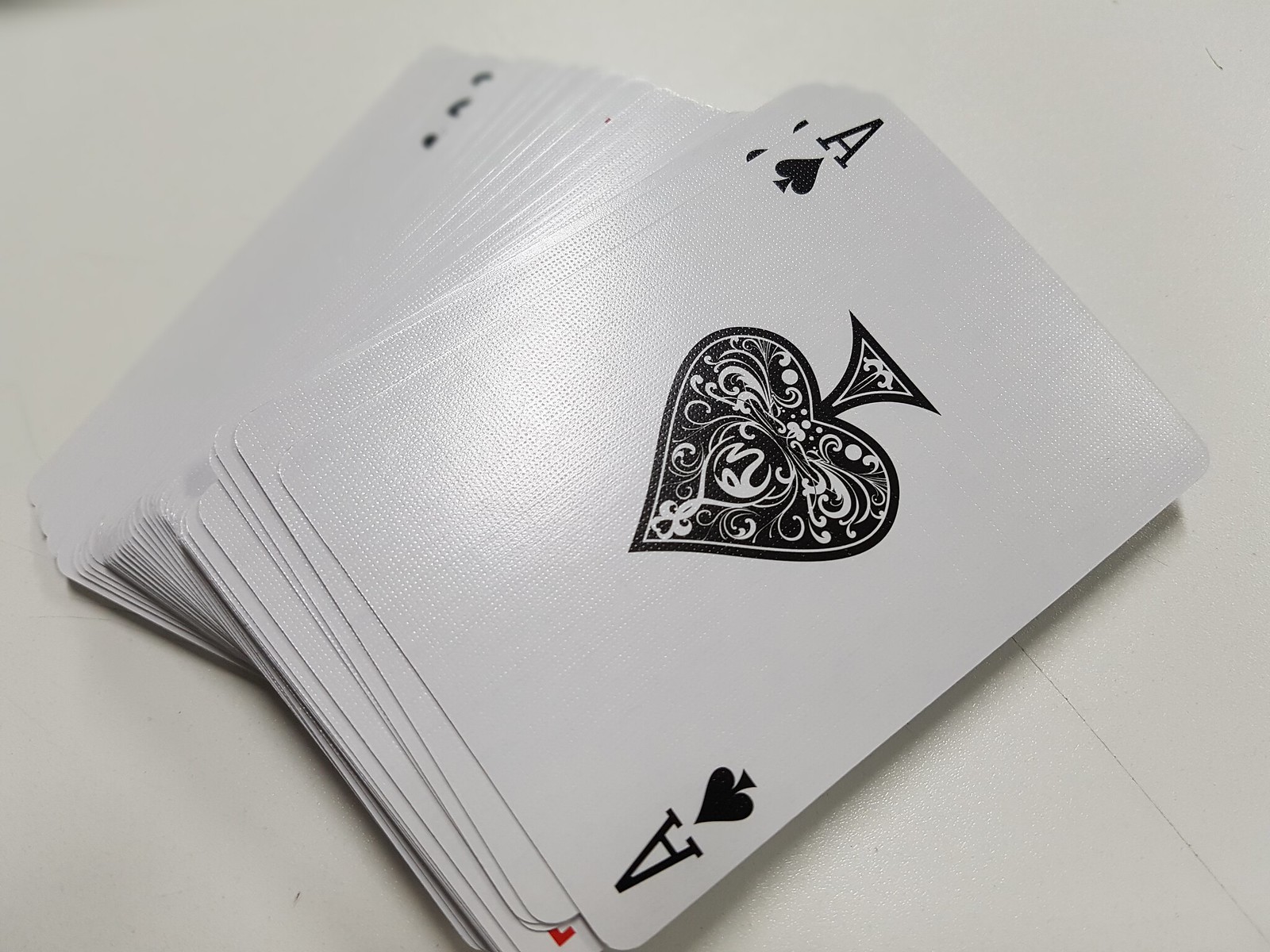A close-up image captures a neatly stacked deck of playing cards on a slightly glossy white tabletop. The vibrant white background enhances the crispness of the cards, emphasizing the clean layout. The deck appears complete, neatly piled in a single stack. Dominating the top of the pile is the Ace of Spades, instantly recognizable by its distinct design. The card features a prominent, large black spade symbol in its center, with a smaller black spade located in the top left and bottom right corners. Accompanying these smaller spades are the letter 'A' in a bold black font, signifying it as the ace. The remaining cards are tightly stacked beneath, their identities hidden from view, contributing to the sense of anticipation and mystery typically associated with a shuffled deck.